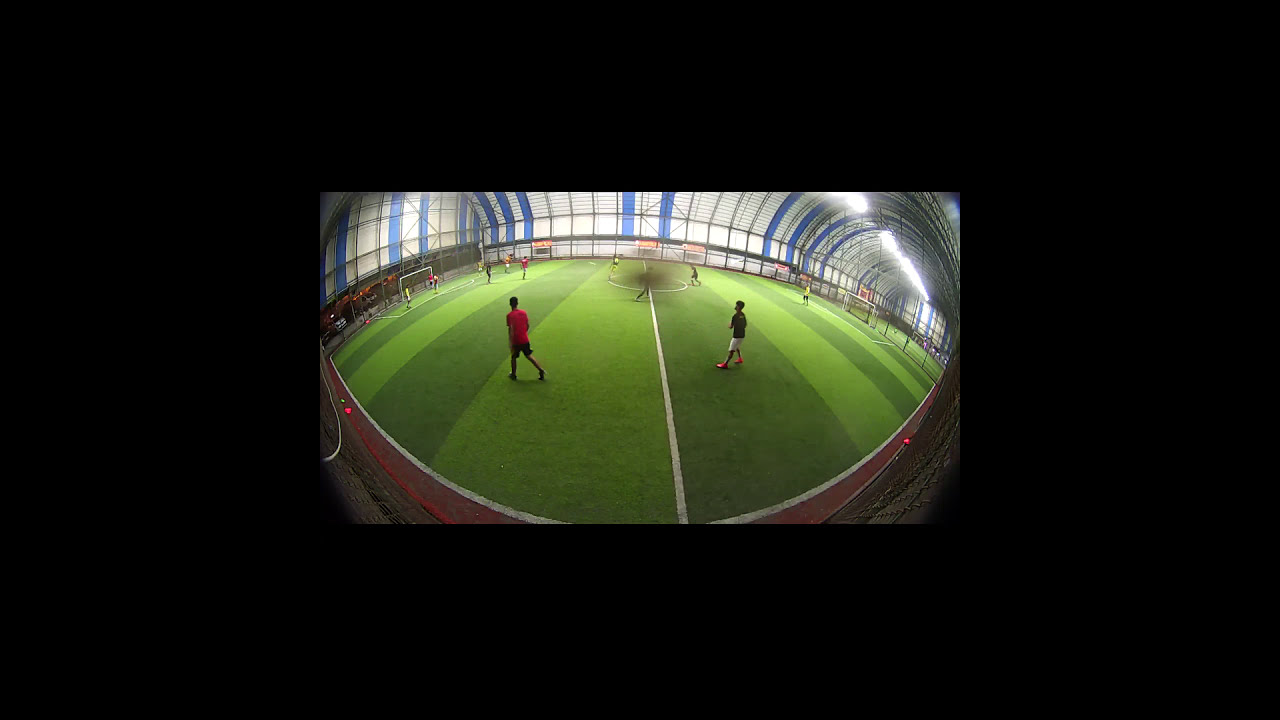The image portrays an indoor soccer field that prominently features a thick black border on all sides, emphasizing the scene in the center. The indoor setting is characterized by a curved roof, enclosing a neatly maintained practice field with alternating light and dark green vertical stripes of grass. A white midfield line bisects the image from bottom to top, suggesting a separation between two practice areas. 

On the left side of the field, a person in a red or orange shirt is walking leftward, while on the right side, another person dressed in a dark shirt and white shorts with bright orange sneakers is also facing left. Both figures are positioned near the midfield line, which extends into the background. In this background, soccer nets and a few more players are visible, though no faces can be seen clearly. The scene lacks any advertising or written elements, focusing solely on the players and the pristine field. Despite the small size and some distortion, the image provides a clear, albeit simple, view of a typical soccer practice environment.